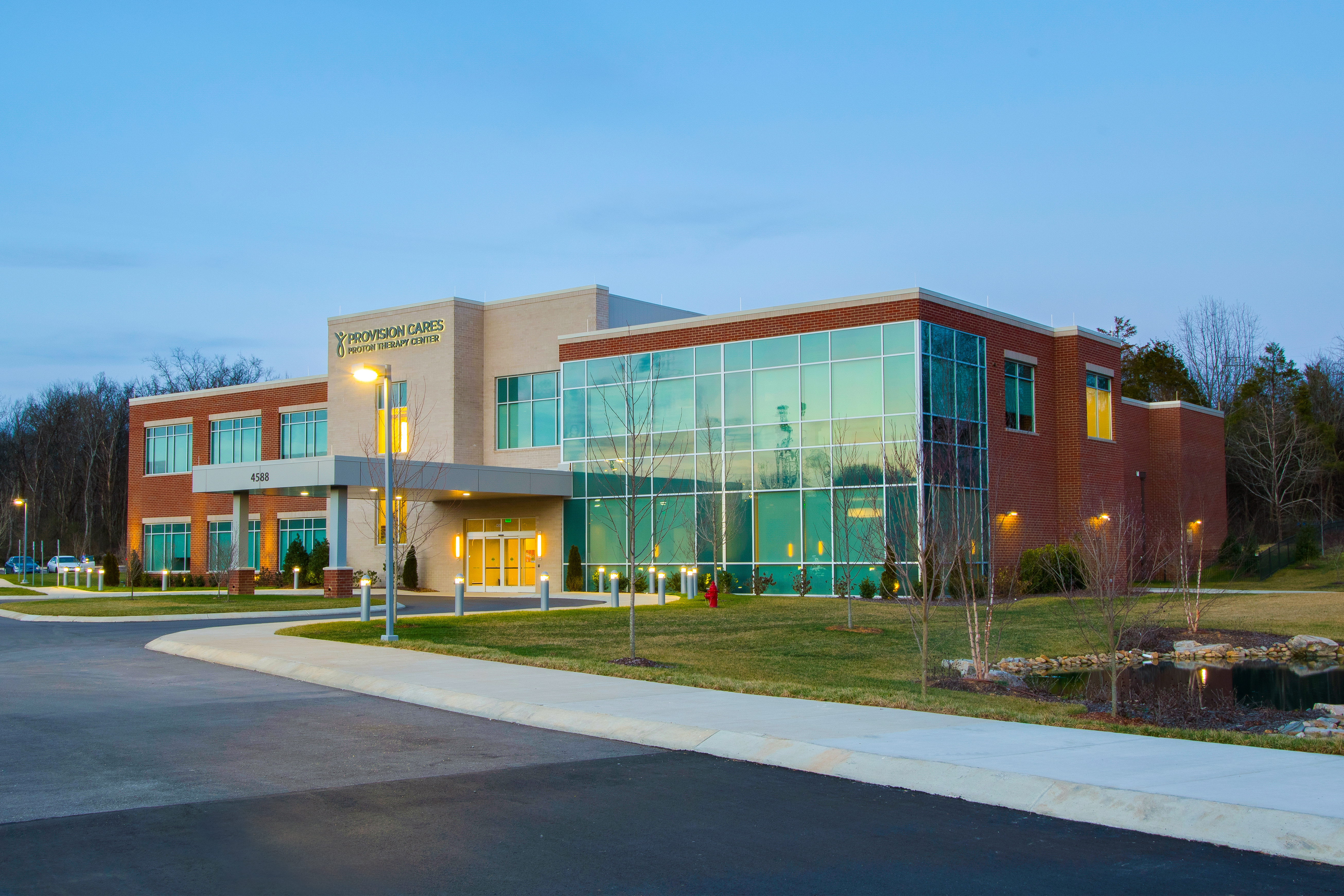This photograph captures an outdoor scene taken in the early dusk hours. The image prominently features the ProVision Cares Proton Therapy Center, a brick building situated in the center-left. The structure boasts wide windows and has its name illuminated at the top, though part of the text is somewhat blurry. The sky above exhibits a dark blue hue, indicative of the approaching evening, with a few patches of clouds adding to the tranquil atmosphere.

The foreground includes a street or driveway area with a sidewalk leading up to the building, flanked by small light poles that illuminate the path. Streetlights are also on, enhancing the setting's twilight ambiance. To the right of the building, near the bottom right corner of the image, a serene pond is visible, bordered by a lush grassy area. Trees form a natural backdrop around the building, adding to the picturesque scene. Additionally, parked cars can be seen to the left of the building in the distance. This detailed landscape merges architectural elements and natural beauty, captured just as day transitions into night.